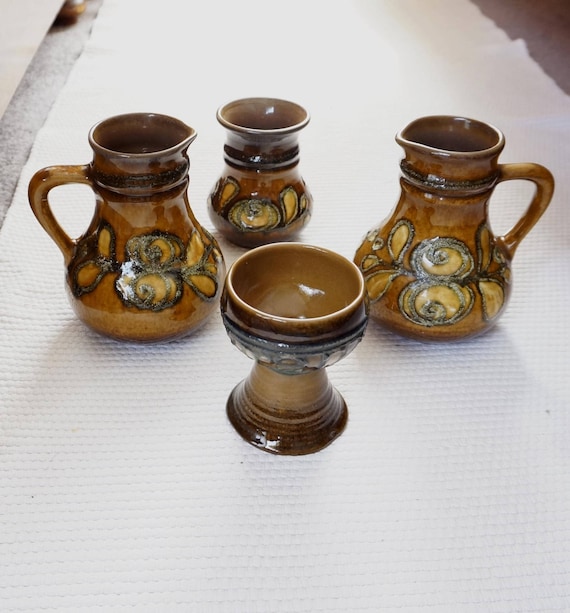The image depicts a white cloth laid out on a table, with a complex arrangement of four antique jars placed on top. The white cloth features a gap with an off-white hue and a brownish-purple section at the top right corner. The jars, which are likely antique stoneware, exhibit a mix of dark brown, light brown, and tan hues, with reflective, shiny surfaces. The first jar in the front resembles a chalice or an open cup with a wide bottom and narrow neck. To the left and right are two large teapot-like pitchers with brown handles and floral designs, possibly used for pouring liquids. The fourth piece, positioned centrally in the back, is a smaller, handle-less version of the pitchers. All the jars have intricate, swirly designs, some with hints of light green detailing, suggesting they were crafted a long time ago but remain sturdy and aesthetically pleasing.